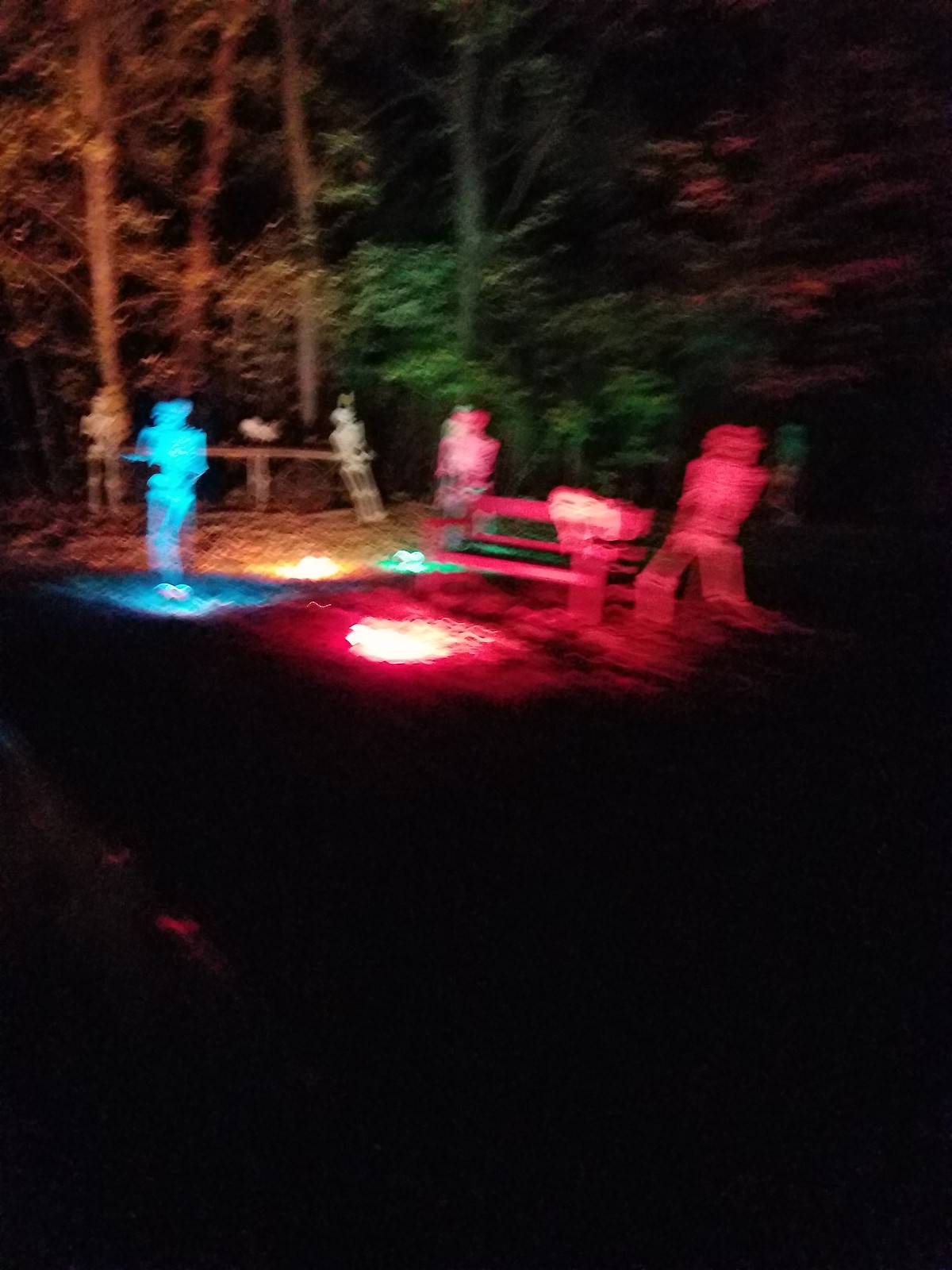A blurry nighttime photo captured from the hood of a moving car, showcasing a park setting. In the background, various colored lights, predominantly red, faintly illuminate four indistinct figures amidst a wooded area. Surrounding trees create a dense backdrop. A barely visible bench suggests a park environment, while a possibly wooden structure leans against what seems to be a wooden fence in the background. The movement of lights and figures indicates activity, all under the quiet canopy of night.